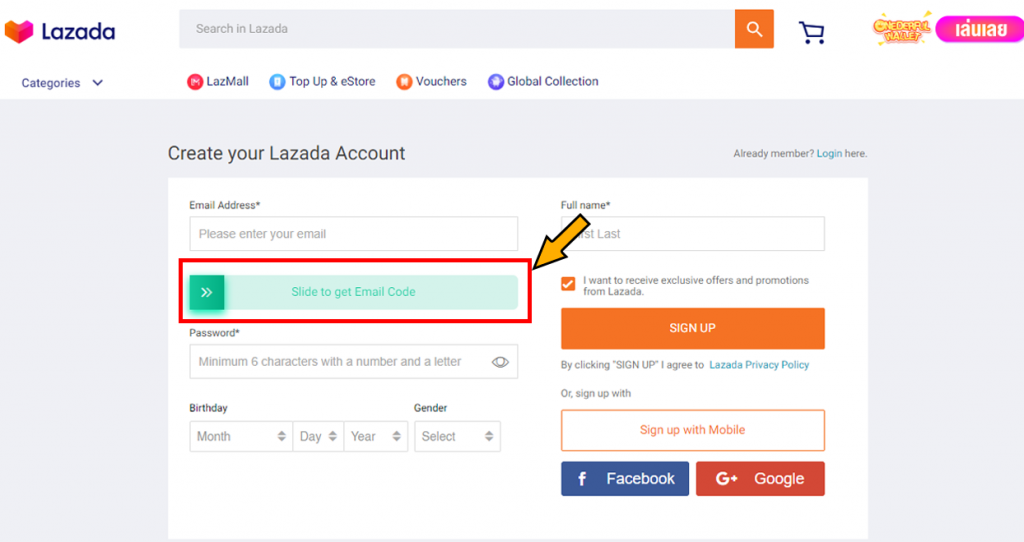A detailed screenshot of the Lazda website interface is depicted. In the upper left corner, the company logo is prominently displayed followed by the name "Lazda." Positioned to the right of the name is a search bar titled "Search in Lazda," accompanied by a magnifying glass icon within an orange button. Adjacent to the search bar on the right, there is a shopping cart icon. Next to this is an icon, possibly representing a digital wallet labeled "Deterol," and an icon or text that reads "Iowa," which could either be in another language or relevant jargon relating to the company's services. 

The primary language of the website content appears to be English. Below the primary navigation bar, there's another menu offering a variety of options: "Categories" is listed first as a drop-down menu, followed by "LazMail," "Top-up and e-stores," "Vouchers," and "Global Collection."

Further down, there is a form dedicated to account creation titled "Create your Lazda account." To its right, there is a prompt for existing users to log in, stating "Already a member? Log in here." The form itself is organized into two columns with fields for entering an email address, full name, password, birthday, and gender. There's also an option to receive exclusive offers or promotions from Lazda via a checkbox. Towards the bottom of the form, users can finalize their registration by clicking "Sign up" or alternatively "Sign up with mobile." Additionally, there are buttons for signing up through Facebook and Google Plus.